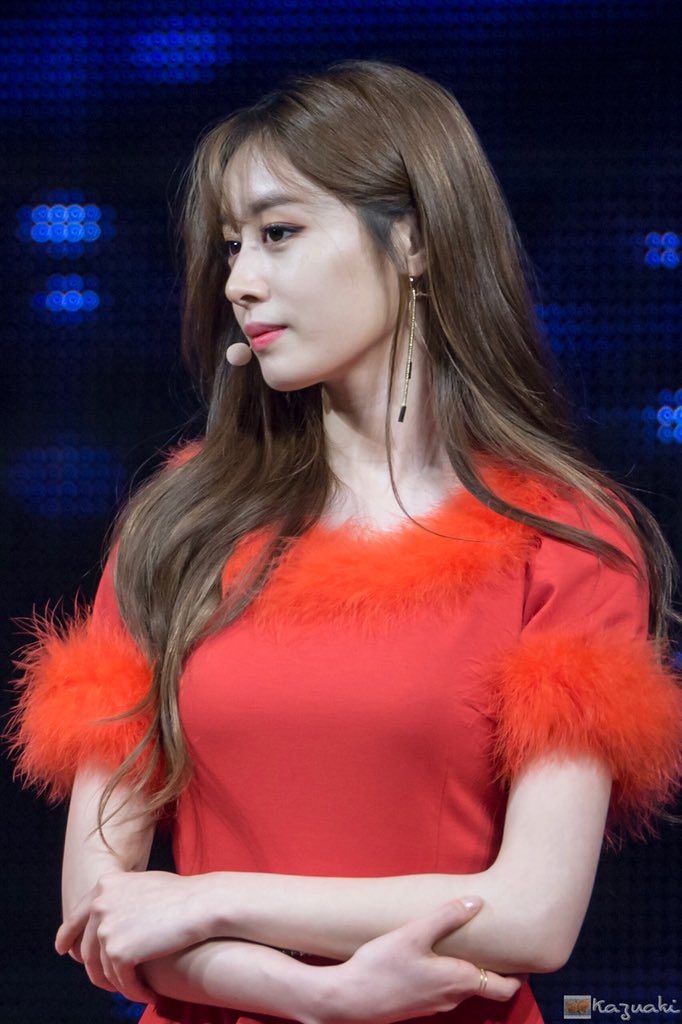In a well-lit photographic image with a dark background illuminated by various blue and neon lights, a young woman, who appears to be of Asian or half-Asian descent, is featured. She has long brown hair cascading past her shoulders and over her chest, adorned with a delicate, string-like earring. The woman is wearing a vibrant red short-sleeve shirt with faux fur trim on the sleeves and neckline. Her arms are crossed in front of her slim frame, exuding a composed yet confident demeanor. She has a microphone positioned in front of her mouth, suggesting she might be recording or performing. While her gaze is slightly downward, she offers a subtle smirk. The illuminated background hints she might be in a recording studio, a concert hall, or a television studio. The photograph bears the text "K-A-Z-U-A-K-I" in the bottom right corner, accompanied by a small red and yellow logo.